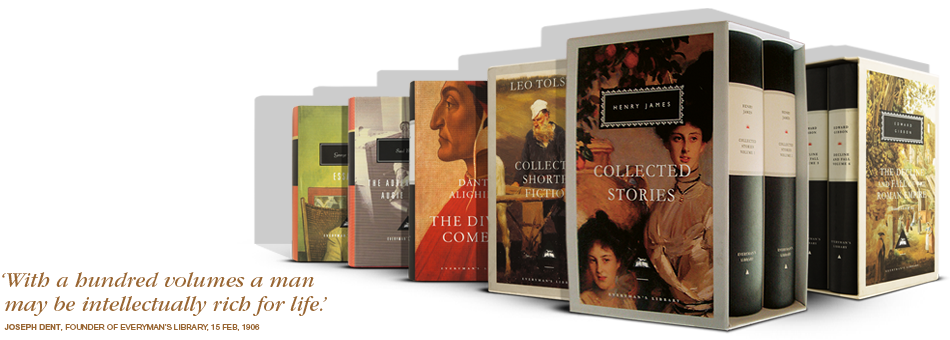The image showcases a meticulously arranged collection of book sets, prominently displayed in makeshift cardboard shelves. Each container has an open side, allowing easy access to the volumes inside. On the left side of the image, a quote by Joseph Dent, founder of Everyman's Library, from 15 February 1906, reads in gold lettering: "With a hundred volumes, a man may be intellectually rich for life." On the right side, there are several black-covered books, each adorned with white labels. The front-most set, consisting of two books bundled together, is titled "Collected Stories." The cover illustration features two women in vintage antique clothing, one standing on the right and the other situated at the bottom left. Additionally, there is a visible set by an author with the last name partially spelled, "Leo Tols," indicating another collection of classic literature, further emphasizing the intellectual richness these volumes offer.